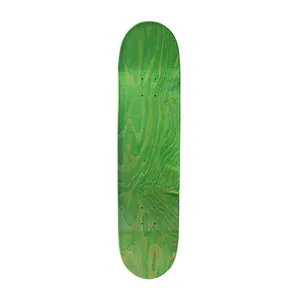The photograph features a simple composition with a completely white background, highlighting a centrally placed, elongated, ovoid-shaped green object that resembles a stretched-out oval or a wide nail file. This green shape, reminiscent of a band-aid, displays a mottled, gradient texture, transitioning from darker green at the top to lighter green in the middle, and then returning to a darker green towards the bottom, with faint yellow designs interspersed throughout, giving it a watercolor effect. The object is subtly shiny, suggesting a textured, painted surface with an appearance of unsmoothed paint. At both the top and the bottom of this vertically oriented item are four small dots, arranged in a square pattern, totaling eight holes to aid breathability. Wrinkles on the surface hint at a material that might be paper or rubbery.